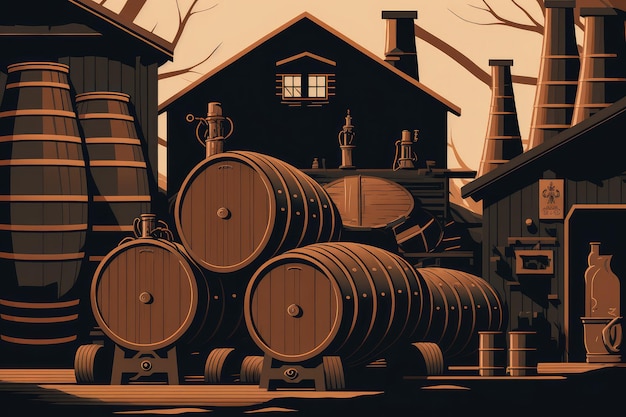The image is a computer-rendered or painted scene in predominantly brown and dark gray tones. The backdrop features a sky with a tan or beige hue, against which a cluster of buildings is set. These structures, appearing to be made of dark gray charcoal or brown wood, are accented with tall kiln-like chimneys. The central building, likely two stories with high windows and a chimney, resembles a garage or workshop. 

In the foreground, numerous large wooden barrels, some with tan rings, are positioned on their sides atop wooden carts or stands, suggesting storage or transport. Additionally, several barrels stand upright to the left, while a few metal cylindrical drums are visible to the right. A smaller shed-like building with possible glass jars and signage stands beside the main structure. Scattered around the scene are more barrels and jars, lending the atmosphere a rustic, industrial feel. The background subtly hints at tree branches framing the edges, completing the detailed, monochromatic composition.